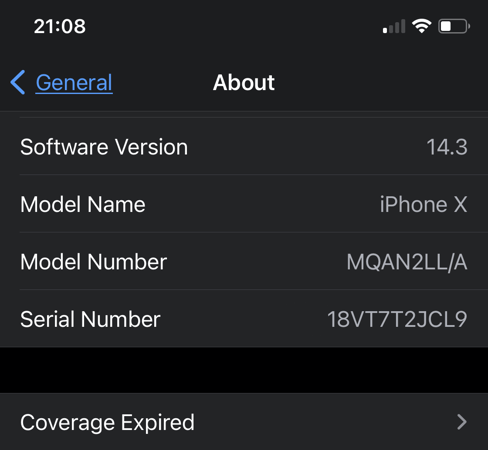The image displays a detailed information page for an iPhone X, showcasing essential device details against a black screen with predominantly white text. The headings include "Software Version 14.3," "Model Name: iPhone X," "Model Number: MQAN2LL/A," and "Serial Number: 18VT7T2JCL9." At the top of the screen, the time is displayed as 21:08. A blue button labeled "General" with a left-pointing arrow provides access to more general information about the device. At the bottom, there is an icon with a right-pointing arrow next to the heading "Coverage Expired," indicating the device's expired warranty or support coverage and hinting at renewal dates. Overall, the page offers a comprehensive summary of the iPhone X's specifications and status.